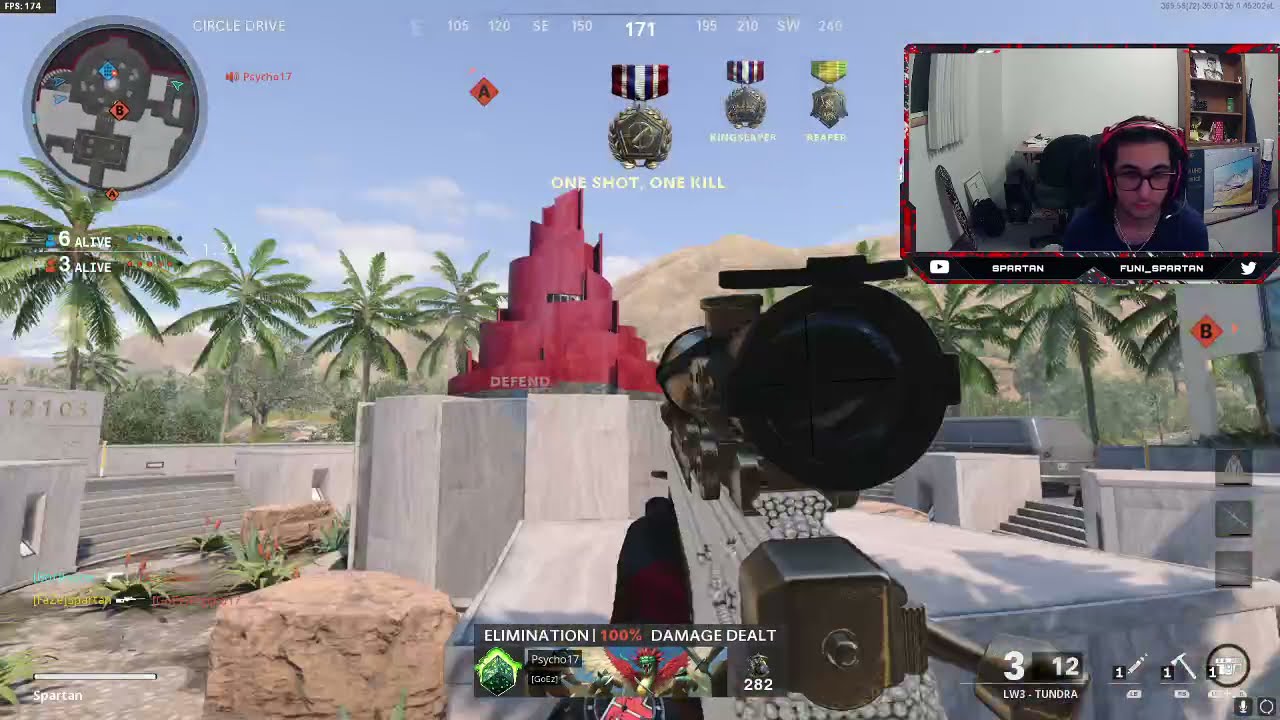This detailed screenshot from a first-person shooter video game depicts a desert environment with scattered, tall palm trees and distant arid mountains, set against a blue sky filled with white clouds. Central to the scene is a white compound topped with a red statue on a tall round pillar, surrounded by rocks and boulders. In the game view, a rifle with a scope is visible, held by a hand wearing a black glove.

The upper section of the image is filled with various in-game elements: medals, with the central one clearly reading “One Shot, One Kill,” while others are less legible but include “Reaper.” To the left is a circular mini-map, shaded in dark and light gray, showing location indicators. Floating text on a red tower within the compound reads "defend."

On the top right, there is a streamer's live feed displaying a man with short hair, black-rimmed glasses, red headphones, a silver necklace, and a dark blue or black t-shirt. The streamer sits in a room, visible next to a bookshelf, gaming from his chair labeled "Spartan." He appears to be playing from a white room with various elements identifiable in the background.